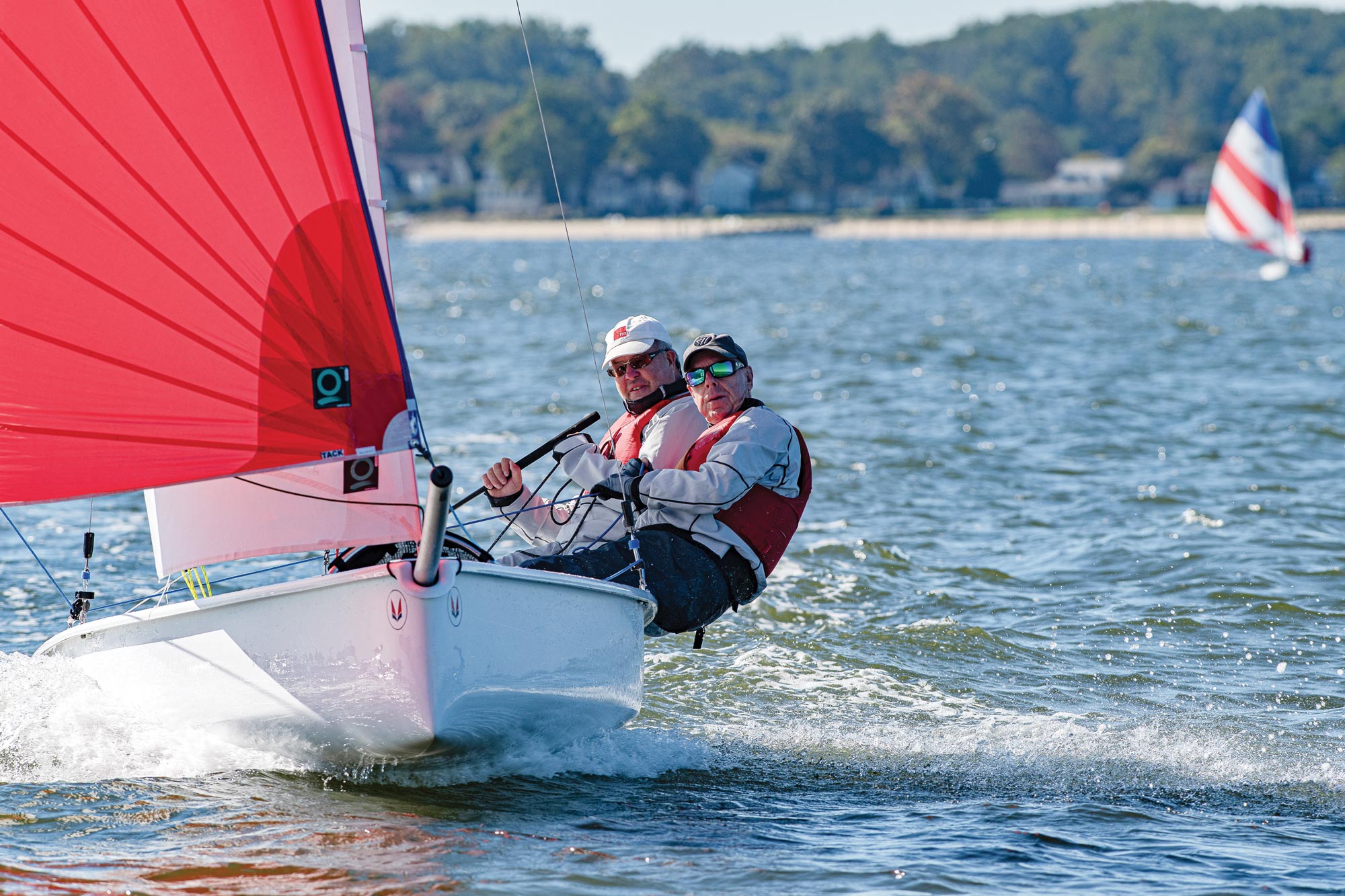In the image, two men are depicted hanging onto the latches on the right side of a white sailboat with a red and semi-transparent sail. The sailboat is cruising on a body of water that could be a lake or the ocean. Both men are dressed similarly in white jackets, red life jackets, and sunglasses. The man toward the front, right side of the boat wears a black cap and black pants, while the man beside him on the left wears a white cap with his pants color not specifically mentioned. In the background, there is a blurred-out scene featuring a dense collection of green trees and some indication of hills and houses along the shore. Another sailboat with a red, white, and blue themed sail is visible to the right, adding more context to the water scenery. The overall focus of the picture is these two men and their sailboat, with land and other elements providing a scenic backdrop.